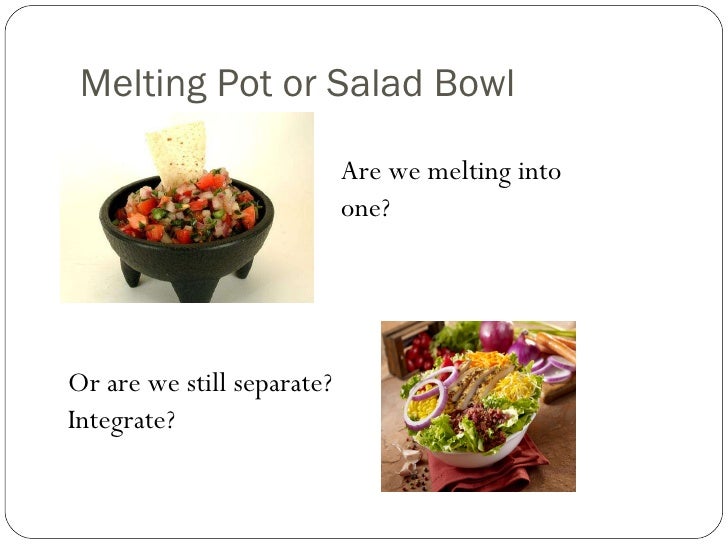The image is a color slide featuring two photographs framed by a large white rectangle with slightly curved black-lined borders, surrounded by black text. The caption at the top reads "Melting pot or salad bowl. Are we melting into one or are we still separate? Integrate." The top left photograph depicts a black bowl with built-in legs, filled with chopped tomatoes, green plants, and onions, with a triangular white tortilla chip protruding from the mixture, resembling a salsa dish. The bottom right photograph shows a large white bowl containing a fresh garden salad, topped with chicken, cheese, and various vegetables. The vibrant colors in the image include red, green, white, tan, yellow, purple, burgundy, brown, and orange, highlighting the diverse elements within each bowl.